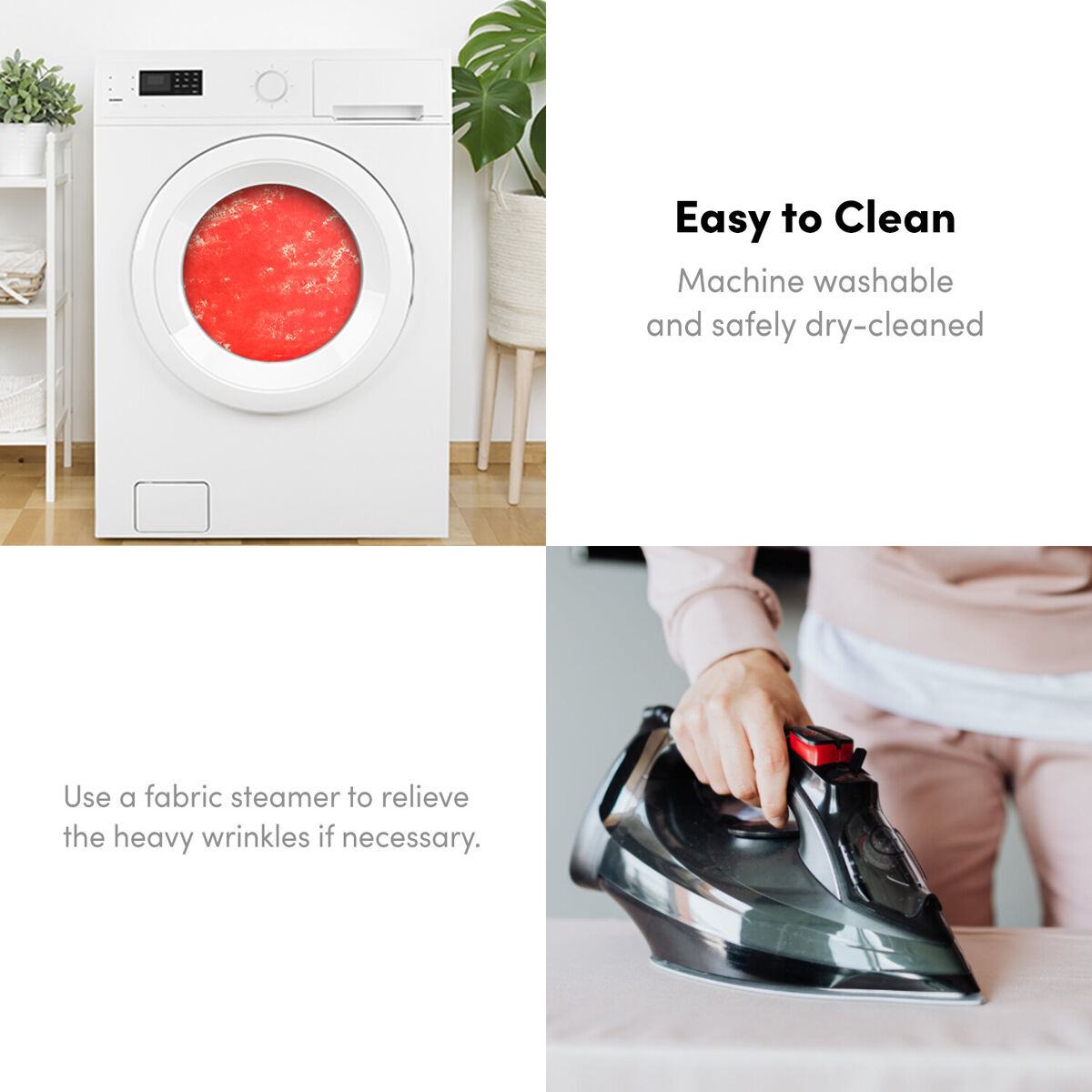In this image, there are two photos placed side by side. The top left photo depicts a white front-loading washing machine on a white background. Visible through the machine's clear circular door is an orange item, possibly a sheet. To the right of the washing machine is a large planter on wooden legs with big green leaves, while to the left, a two-shelf stand holds a smaller potted plant with additional shelves below it. Prominently displayed text next to the machine reads, "easy to clean, machine washable and safely dry cleaned."

The bottom photo shows a woman’s hand ironing a white fabric with a silver and black steam iron featuring a red button. The person, dressed in a pink sweatsuit with a white shirt underneath, is using the iron to smooth out wrinkles. Accompanying text advises, "use a fabric steamer to release the heavy wrinkles if necessary."